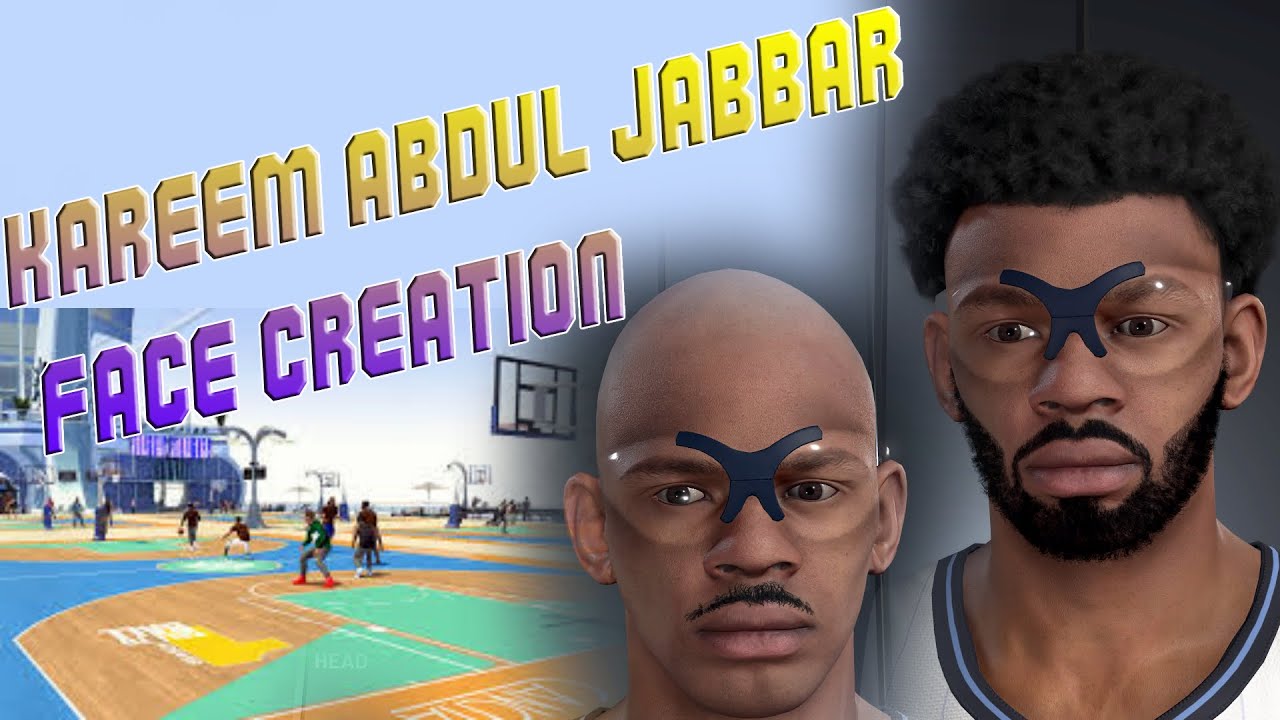The horizontally oriented image showcases a computer-generated graphic depicting legendary NBA players from the past. In the background, a blue sky transitions gently to white near the horizon, creating a slight ombre effect. The sky is otherwise a consistent flat blue, except for the fading near the horizon. Several elements such as billboards or stadium structures and basketball hoops suggest the setting of an outdoor basketball court.

In the bottom left corner, the blue, brown, and green court is marked with white lines. The scene features computer-generated male basketball players engaged in a game. One player, clutching the ball, is being guarded by others.

Dominating the upper and bottom right sections, two prominent African-American players are illustrated. The first player, partially visible up to his chin, is bald, with a black mustache and glasses that appear to have black tape over his eyebrows and nose. He gazes slightly to the side.

Next to him stands a taller player with afro hair, a beard, and a mustache, wearing similar glasses. More of his white jersey with bluish accents is visible, prominently displaying the name "Kareem Abdul-Jabbar" in large, yellowish letters. The positioning and size of the players draw significant attention, anchoring the middle and right side of the image.